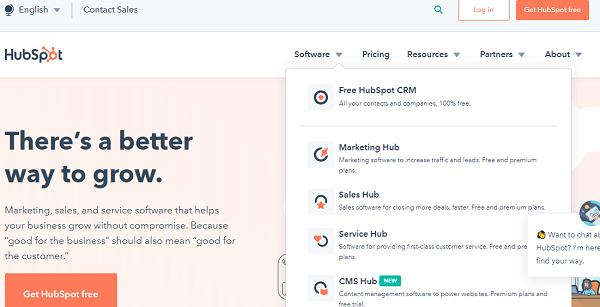The image is a detailed screenshot of a HubSpot webpage. In the top left corner, there's the word "English" accompanied by a globe icon, followed by the "Contact Sales" option. In the top right corner, there are links for “Get HubSpot Free,” “Login,” and a magnifying glass icon indicating a search function.

Following downwards from the “English” option on the left, there's the HubSpot logo. To the right of the logo, there's a navigation menu that reads "Software" with a downward arrow. Hovering over this reveals a drop-down menu featuring options like "Free HubSpot CRM," "Marketing Hub," "Sales Hub," "Service Hub," and "CMS Hub." 

To the right of the "Software" menu item, the navigation continues with "Pricing," "Resources" (with a downward arrow for more options), "Partners" (also with a downward arrow), and "About" (again with a downward arrow). 

Further down on the left side of the pop-up tab, there’s a prominent message that reads "There's a better way to grow." It is followed by a description: "Marketing, sales, and service software that helps your business grow without compromise because good for the business should also mean good for the customer." The call-to-action "Get HubSpot Free" is highlighted.

In the top right area, there’s an image of a person seeming to sit in a chair. At the bottom right of the image, there's a small robot icon with a chat prompt that says “Want to chat?” Next to it, there’s text that reads "HubSpot, I'm here. Find your way."

This detailed description aims to capture every element visible in the image, providing a clear and thorough understanding of the webpage layout and content.